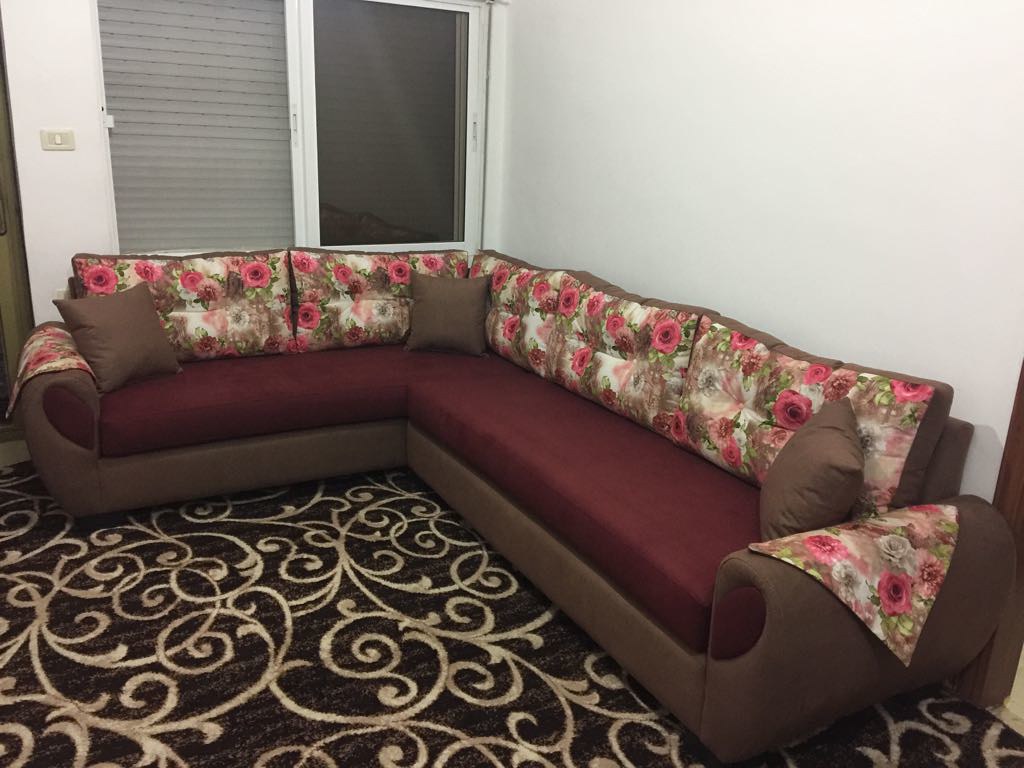The image captures a meticulously designed living room featuring a cozy L-shaped sectional couch positioned in the corner of the room. The room itself is enveloped in white walls, enhancing the brightness and spaciousness of the space. The sectional sofa's base is a rich chocolate brown, while the cushions above are a deep maroon, adding warmth and comfort. The sofa is adorned with floral back pillows showcasing intricate designs with white and pink flowers alongside green foliage, and three smaller, square chocolate brown throw pillows strategically placed—one at the corner and two at the ends of the sectional.

Behind the couch, on the left side, there is a door or possibly a window fitted with gray blinds drawn up, while on the right side, darker blinds cover an adjacent window, giving an impression of nighttime darkness. The armrests of the couch feature doilies with matching floral patterns, adding a quaint, homely touch.

Dominating the floor is a large, black carpet that provides a striking contrast against the lighter elements of the room. The carpet is adorned with elaborate white swirls and floral designs, lending a vintage feel to the space. The intricate patterns on the carpet converge with those on the throw pillows, creating a cohesive and aesthetically pleasing look throughout the living room.